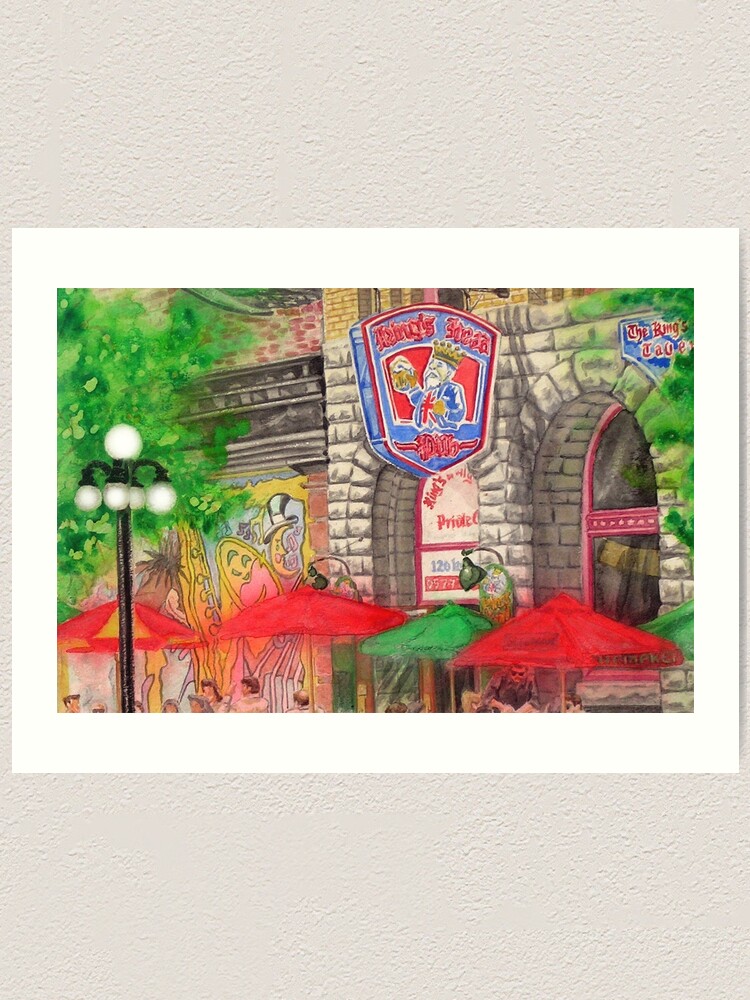The image in question appears to be a detailed scan of a greeting card featuring a colorful computer-enhanced illustration with a distinct medieval theme. The card itself is beige with a mottled texture and houses a central, rectangular picture outlined in white. The focal point of this image appears to be a façade reminiscent of an old European pub or castle wall, possibly depicting an exterior scene rich in historical ambience.

This plausible medieval castle scene showcases gray stone walls with two imposing archways leading inward. Above one of the arches, a neon sign hangs. The sign features an image of a king with a white beard, wearing a yellow crown, a blue robe, and a red cross on his chest. This king figure, raising a beer stein to his mouth, suggests the name "King’s Head South," though the text is sharply blurred.

In the foreground, red and green merchant stalls line the bottom of the scene, where modern people—some donning button-down shirts and sunglasses—sit under vibrant umbrellas. The juxtaposition of the old and the new is accentuated by a black street lamp with a white globe on top and four smaller globes around it, which stands prominently to one side of the scene. Flanking either side of the image are green-leafed trees, adding a touch of nature to the vividly colored, slightly smudged drawing.

The entire illustration sits against what appears to be a gray wall with a light popcorn texture, adding depth to the indoor photograph of this historically evocative yet modernly portrayed scene.